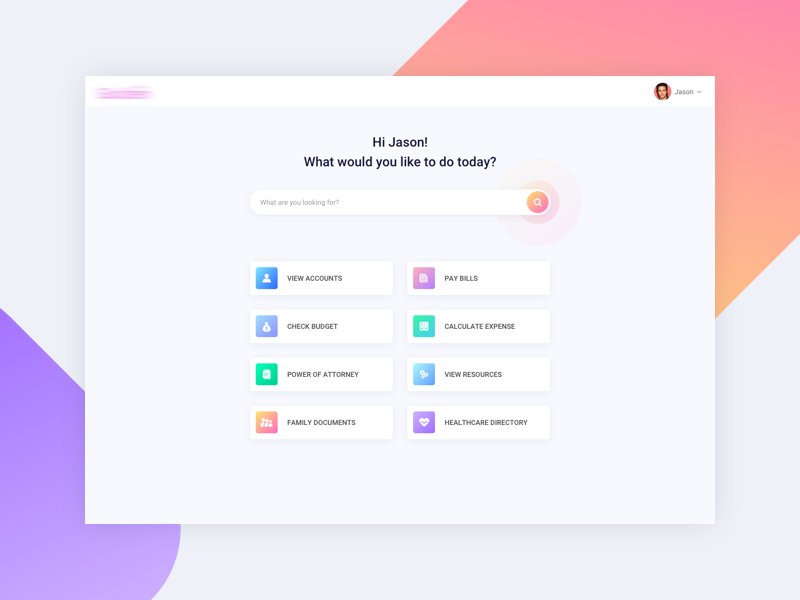The desktop screenshot features a beautifully designed background that blends light gray, light purple, and light pink with subtle gradients of light orange, creating a serene and visually appealing canvas. 

Dominating the center is a distinct, square-shaped cutout where the UI elements are displayed. In the top-left corner of this cutout, there's a blurred image featuring the company’s name. Adjacent to this, on the right, is the user’s information with the name "Jason" prominently displayed. Alongside Jason's name is a circular avatar of him, accompanied by a drop-down button to its right.

Below the user's name is a friendly greeting text, "Hi Jason, what would you like to do today?", inviting interaction. Just beneath this message is a sleek, white pill-shaped search bar with the placeholder text, "What are you looking for?" On the right end of the search bar, there’s a spherical magnifying glass icon used to trigger the search functionality after the user enters their query.

Further down, the interface is organized neatly into two columns with a total of eight functional divisions, each housed in its own rectangular box. 

**First Column:**
1. **View Accounts:** Displayed with a corresponding colored square icon.
2. **Check Budget:** Accompanied by its own unique colored square icon.
3. **Power of Attorney:** Marked with a relevant colored square icon.
4. **Family Documents:** Presented with an associated colored square icon.

**Second Column:**
1. **Pay Bills:** Identified with an appropriate colored square icon.
2. **Calculate Expense:** Denoted by its respective colored square icon.
3. **View Resources:** Linked with a matching colored square icon.
4. **Healthcare Directory:** Characterized by its distinct colored square icon.

The clean layout and intuitive design ensure quick access and ease of use, making this a highly functional and user-friendly interface.